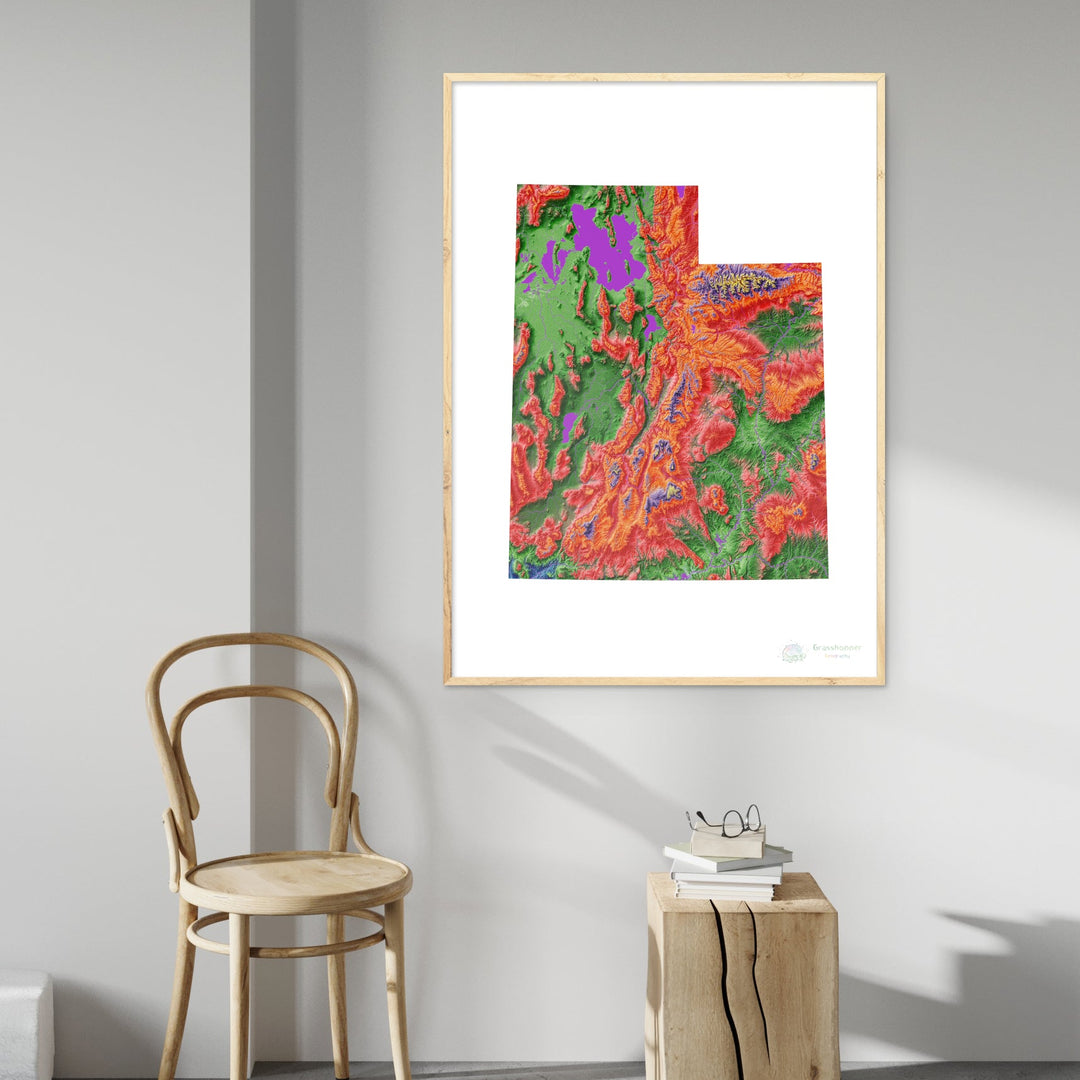This color photograph, taken indoors, showcases a room with a gray-painted wall bathed in streaming sunlight, casting distinct shadows. The main focus is a piece of artwork hanging on the wall, framed in a light blonde wood. The artwork itself has a white matte background and features a brightly colored abstract image resembling a Tetris block or an L-shape, evoking the topography of Utah. The vibrant ink blocks encompass shades of purple, red, green, orange, and hints of yellow. Beneath the artwork is a wooden table with a natural finish, on which rest a stack of four books topped with a pair of eyeglasses. To the left of the table stands a solid wooden chair, similar to a barstool but with a backrest, also casting its shadow on the wall.​​